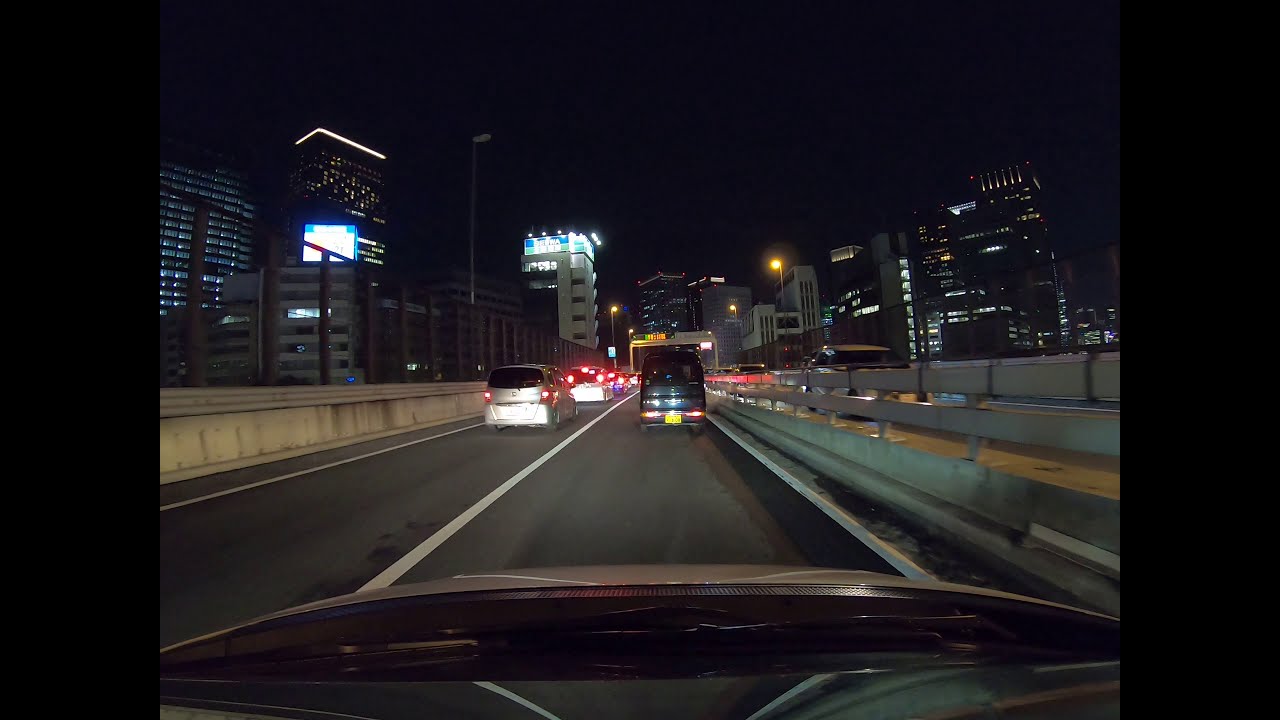The image is a nighttime photograph taken from the perspective of someone driving on a congested highway, possibly in Tokyo. The scene is outdoors, illuminated by various colored lights including black, white, gray, red, yellow, orange, blue, and pink. The photo shows the dark metal front bumper of a car at the bottom, with a dark gray road extending up towards the center. The road features white lane markings and is flanked by gray concrete medians. Numerous vehicles, likely stuck in traffic, are visible; their red brake lights indicate the slow pace. The sky is black, and the tall high-rise buildings on either side of the road are lit up with sparkling lights in their windows and on their rooftops. The highway has two lanes in the same direction, with several white lanes creating vertical stripes. Neon signs and illuminated billboards also punctuate the scenery, adding to the urban skyline's glow. The overall ambiance conveys a bustling, brightly-lit city at night.